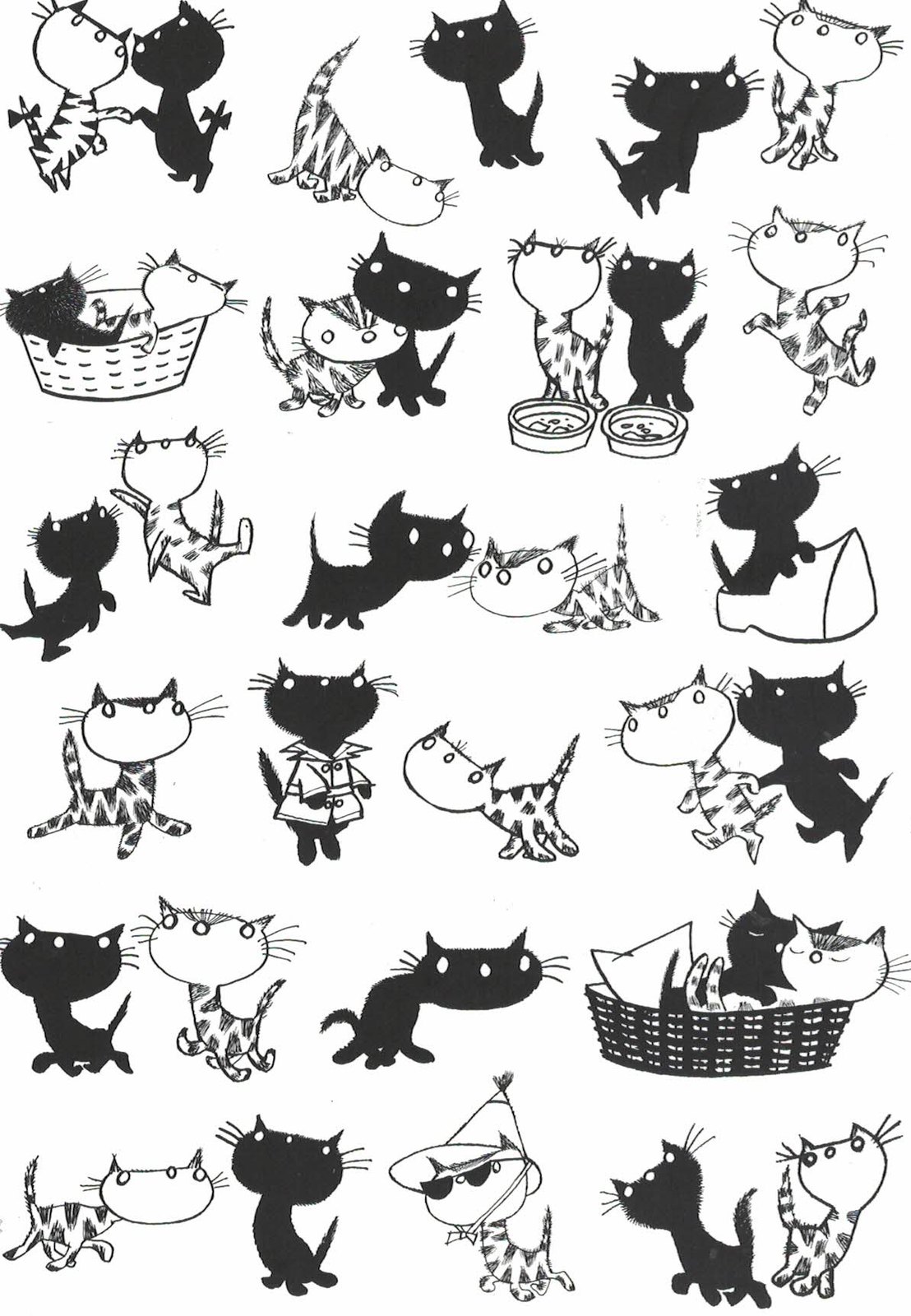The image is an illustration featuring a series of drawings of two cats depicted in various scenarios and poses. There are three columns and six rows, making a total of 18 individual drawings. The cats include a black cat with white eyes, a white nose, and visible whiskers, and a white cat adorned with black stripes.

These detailed sketches capture the cats in multiple interactions and solo moments. They are seen playing and snuggling together, engaged in activities like shaking hands, eating from their separate food bowls, and lying together in a basket. The black cat is illustrated wearing a trench coat in one drawing, while the white cat with black stripes is shown donning a pointed hat in another. There’s also an image where the black cat looks up while the white cat glances back. Individual images include the black cat wearing shades and the white cat appearing alone in different scenes. The background of each drawing remains consistently white, allowing the vibrant and varied poses of the cats to stand out prominently.